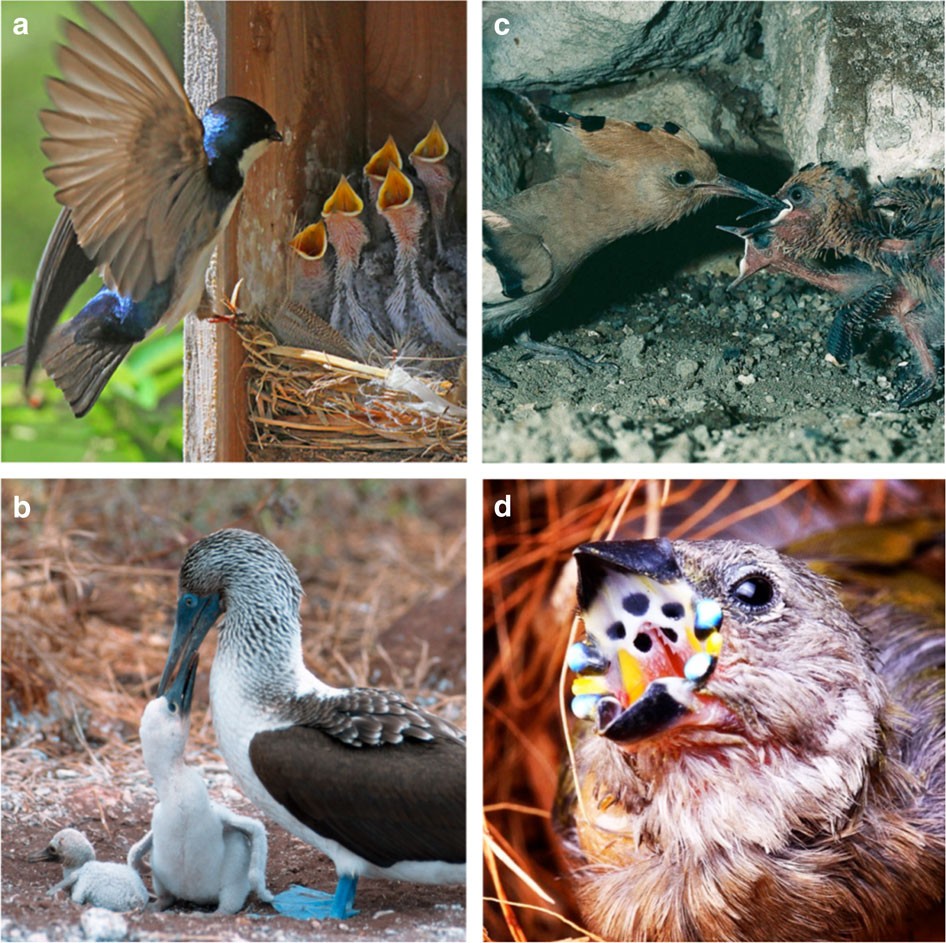The image is a composite of four large, square, colored photographs arranged in a grid, delineated by a white vertical and horizontal line. Each section is labeled with a white lowercase letter: A (upper left), B (lower left), C (upper right), and D (lower right). These images capture various scenes of birds feeding their young in the wild, each exuding its unique, vibrant details.

In section A, a majestic bird, wings fully spread, descends upon a nest filled with five baby birds, each with mouths wide open in eager anticipation. The photograph beautifully captures the landing moment as the mother bird brings food to her offspring, highlighting their outstretched necks and the urgency of their hunger.

Section B beneath it depicts another scene of parental care, where a bird, standing on the ground, feeds one of her young directly, showcasing the nurturing behavior of birds at eye level. The colors are vivid, emphasizing the intimate exchange between the mother and her chick.

Moving to section C, located in the upper right, the image portrays a more stern interaction. A mother bird, with a focused gaze, points her beak toward one or possibly two of her young, seeming to either scold or instruct them. This photograph offers a glimpse into the more disciplined aspects of avian life.

Finally, in section D at the lower right, a bird is shown with its mouth agape, filled with a strikingly colorful item that includes shades of white with black dots, red, and yellow. This vivid, almost ornamental display within the bird's mouth captures the eye and adds a dramatic flair to the collection.

Each photograph is sharp and clear, allowing viewers to appreciate the intricate details and the distinct behaviors displayed by different bird species in their natural habitats.